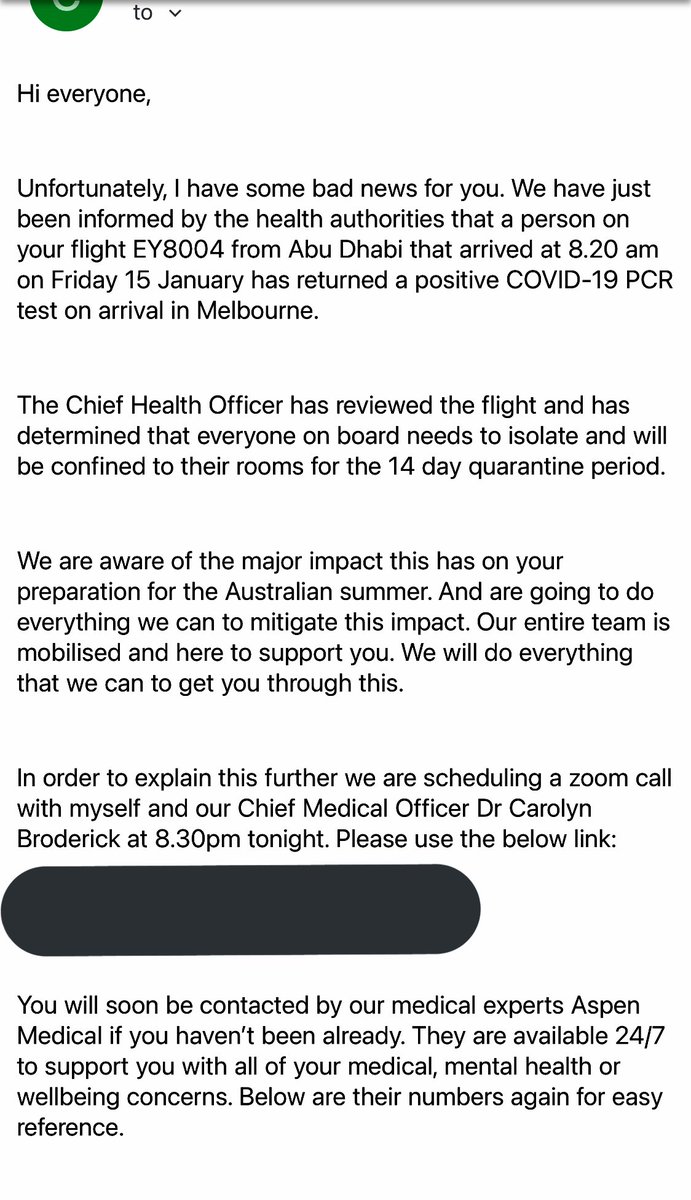**Caption:**

The image features a white background with a light blue print, primarily showcasing a message regarding a COVID-19 update. At the top, there's a small semi-circle design in green with a hint of blue, containing the number "2" with a down arrow.

The message reads:

"Hi everyone,

Unfortunately, I have some bad news for you. We have just been informed by the health authorities that a person on your flight EY8004 from Abu Dhabi, which arrived at 8:20 a.m. on Friday, January 15th, has returned a positive COVID-19 PCR test upon arrival in Melbourne. 

The chief health officer has reviewed the flight and determined that everyone on board needs to isolate and will be confined to their rooms for the 14-day quarantine period. We are aware of the major impact this has on your preparation for the Australian summer and are going to do everything we can to mitigate this impact. Our entire team is mobilized and here to support you. We will do everything that we can to get you through this.

To explain this further, we are scheduling a Zoom call with myself and our chief medical officer, Dr. Carolyn Broderick, at 8:30 p.m. tonight. Please use the link below.

You will soon be contacted by our medical experts, Aspen Medical, if you haven't been already. They are available 24/7 to support you with all of your medical, mental health, or well-being concerns. Below are their numbers again for easy reference."

Towards the bottom of the image, there's a large black box indicating additional contact information and support resources.